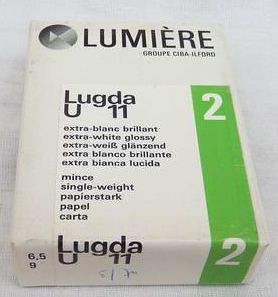The image depicts an up-close, angled photograph of a rectangular package for medication or paper, primarily in white or off-white color. In the top left corner of the package, there is a circle with gradients of gray and white. Just to the right of this circle, “LUMIERE” is printed in black text. Directly below this, the word “G-R-D-U-E-E,” “C-I-N-A,” and a line of unreadable text can be found. 

On the left side of the image, there is another text block that reads “LUGDA,” followed by a “U,” and the number “11.” Below this, it reads “Extra Blanc Brilliant,” followed by several translations of “Extra White Glossy” in different languages. On the right-hand side of the package, a thick green stripe runs vertically down, with the number “2” prominently displayed at the top and another white “2” continuing along the border onto the side of the package.

This photograph captures the details of the packaging, showing both the front and part of the side, and the package is placed on a black marble countertop.